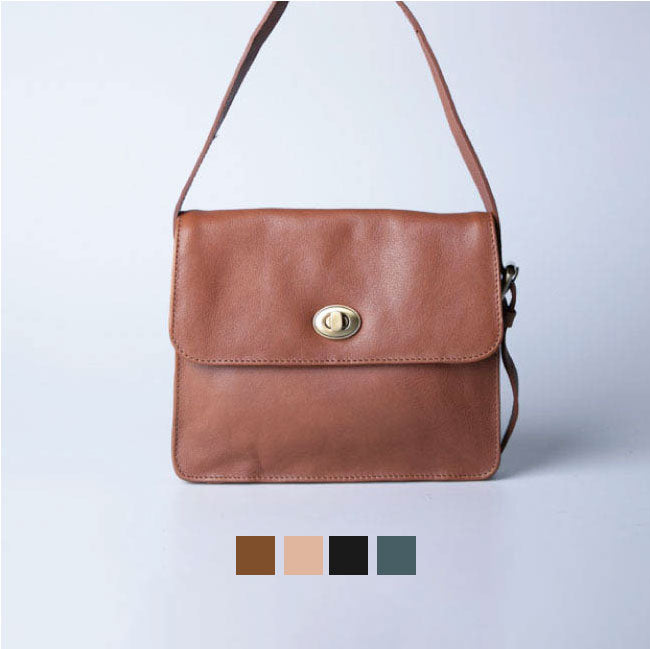This product photograph showcases a rectangular brown leather purse designed for commercial listings such as online shops, catalogs, or websites. The purse features a single flap, secured by an oval-shaped gold clasp on the front. The strap, which arches gracefully above the purse, is connected to silver buckles on both the right and left sides of the bag. The photograph is set against a light gray background, enhancing the focus on the purse. The well-adjusted lighting creates a subtle shadow to the right of the product. Below the purse are four colored squares indicating its availability in multiple colors: the featured brown, tan, black, and a light teal greenish-blue. The purse's elegant design and variety of color options are prominently displayed, making it the focal point of the image.